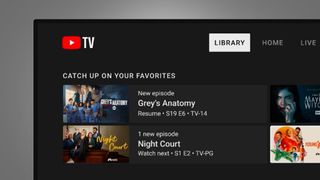This image is a detailed screenshot of the YouTube TV app interface in dark mode. The 'Library' tab is selected, and additional navigation options such as 'Home' and 'Live' are present. Prominently displayed under the 'Library' tab is the suggestion to "Catch up on your favorites". Below, a new episode is available for a show listed as "Season 19, Episode 6", rated TV-14, and an option to resume watching is provided. Directly underneath is "Night Court," indicating one new episode available to watch next, "Season 1, Episode 2," rated TV-PG. To the right of these listings, there are thumbnails for two additional titles; one appears to be a horror movie, while the other seems to be an action-adventure film, possibly reminiscent of "Jumanji" or a travel adventure movie. The viewer's diverse media tastes are highlighted by the variety of genres, ranging from medical drama to sitcom, horror, and action-adventure, although the details on these last two entries are partially obscured.